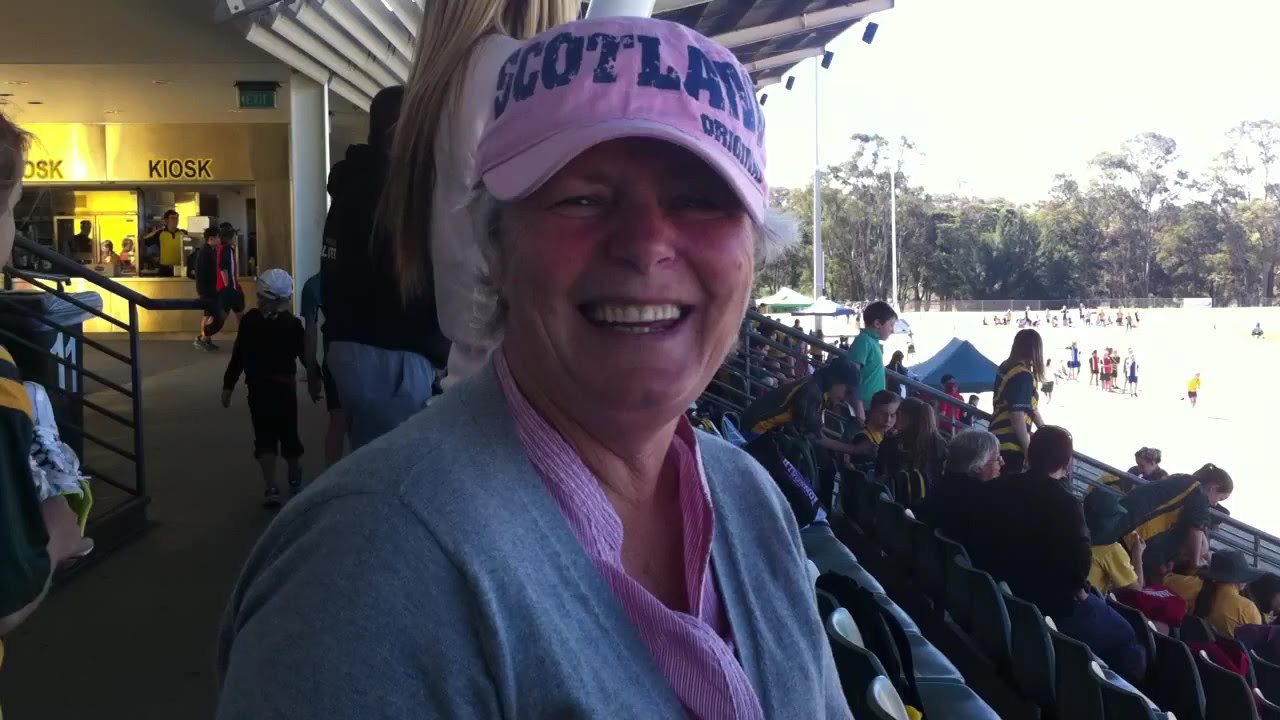The image captures a vibrant scene at a sporting event, focusing on an older woman with gray hair who is smiling warmly and looking forward. She is wearing a blue sweater over a purple and white striped button-up blouse, and on her head is a purple hat that partially reads "SCOTLAN" with the word "original" in smaller letters beneath it. The seating area is covered by a canopy, giving a sense of shelter to the audience. To the left of the image, there is a kiosk with several employees dressed in yellow and black polo shirts standing behind a glass window, ready to serve attendees. The sky above is predominantly gray, providing a neutral backdrop to the lively scene. In the lower right of the image, there are bleachers with people watching the event. The background reveals additional details like trees, poles, and a fence, along with a set of stairs marked by a railing, contributing to the dynamic environment of the venue.